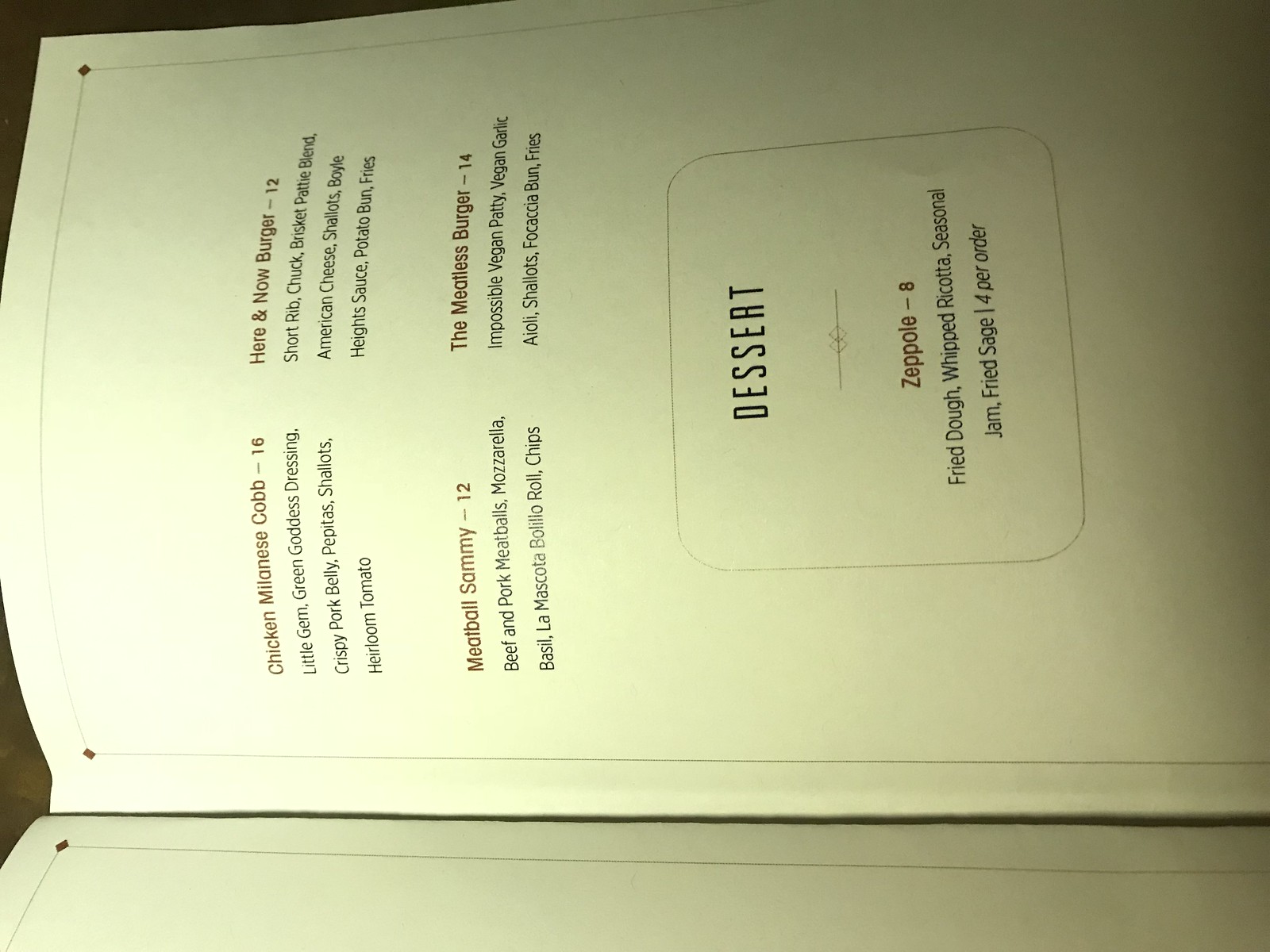This image depicts a detailed page from a restaurant menu, laid horizontally and capturing two partially visible pages. The main page showcases various food items and their respective prices. 

The upper section of the page lists:
- Chicken Milanese Cobb Salad: Priced at $16.
- Meatball Sammy: Priced at $12.

On the right side of the page, the menu continues with:
- "Here and Now" Burger: Priced at $12.
- Meatless Burger: Priced at $14.

At the bottom of the image is a highlighted section dedicated to desserts. This section highlights:
- Zeppole: Priced at $8. Described as fried dough served with whipped ricotta, seasonal jam, fried sage, and notes that four pieces are included per order.

The presentation of the menu items, along with clear pricing and brief descriptions, offers a concise yet comprehensive snapshot of the restaurant's offerings.